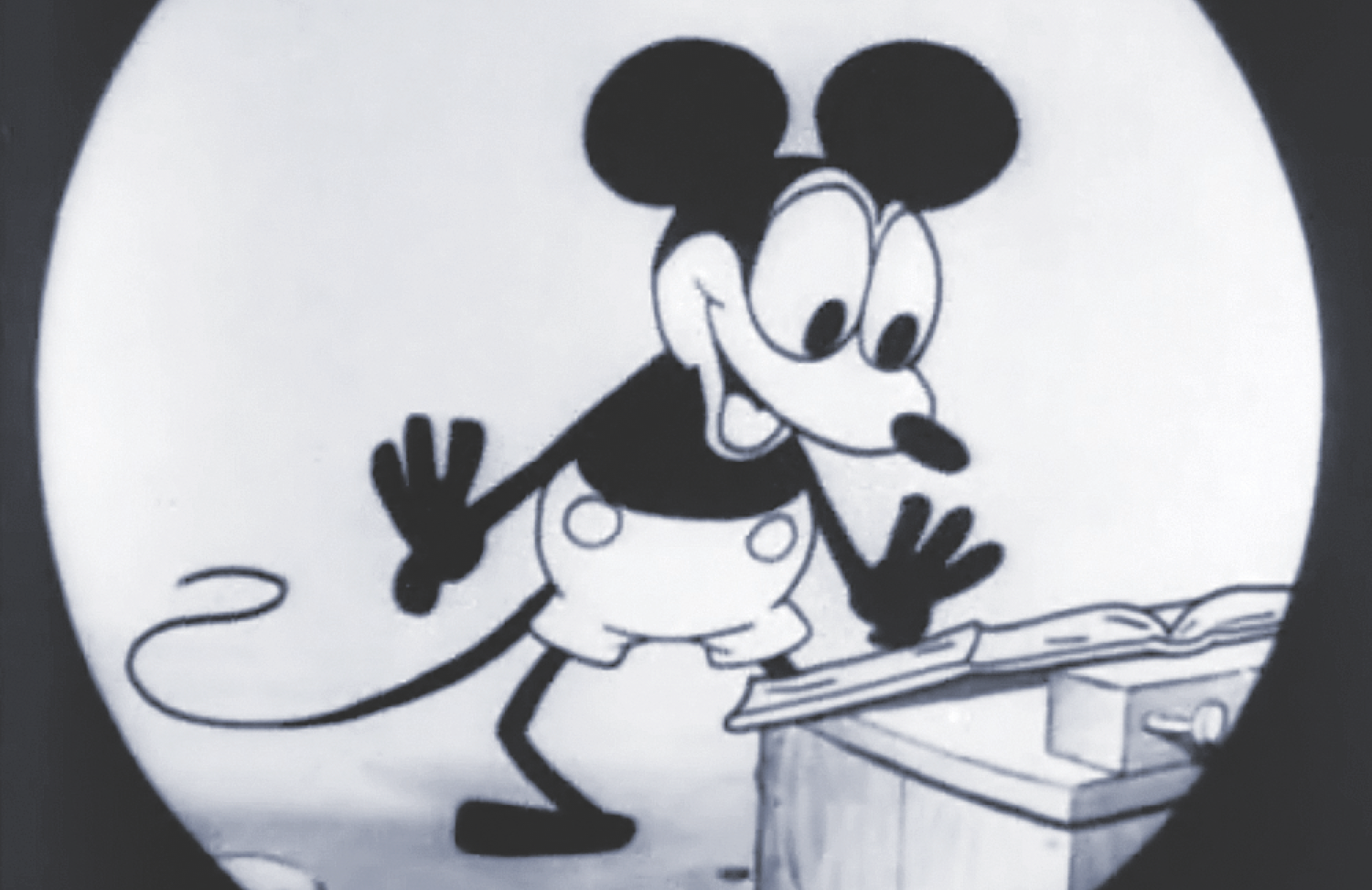This image depicts an early vintage drawing of Disney's classic character, Mickey Mouse, from perhaps one of his earliest cartoons. Mickey is characterized by his entirely black body, including his large, solid black ears, spindly legs, tail, arms, and hands. His face, in contrast, is white with distinctive oval-shaped eyes and a flat, oval-shaped nose. Mickey is shown standing and joyfully reading from an open book placed on a wooden desk. He wears his iconic white shorts adorned with two circular buttons on each side. Mickey's mouth is open in a slight smile, conveying his happiness or surprise at the book's contents. The scene is set against a circular lens focus, highlighting Mickey as the central figure in this nostalgic, black-and-white portrayal.